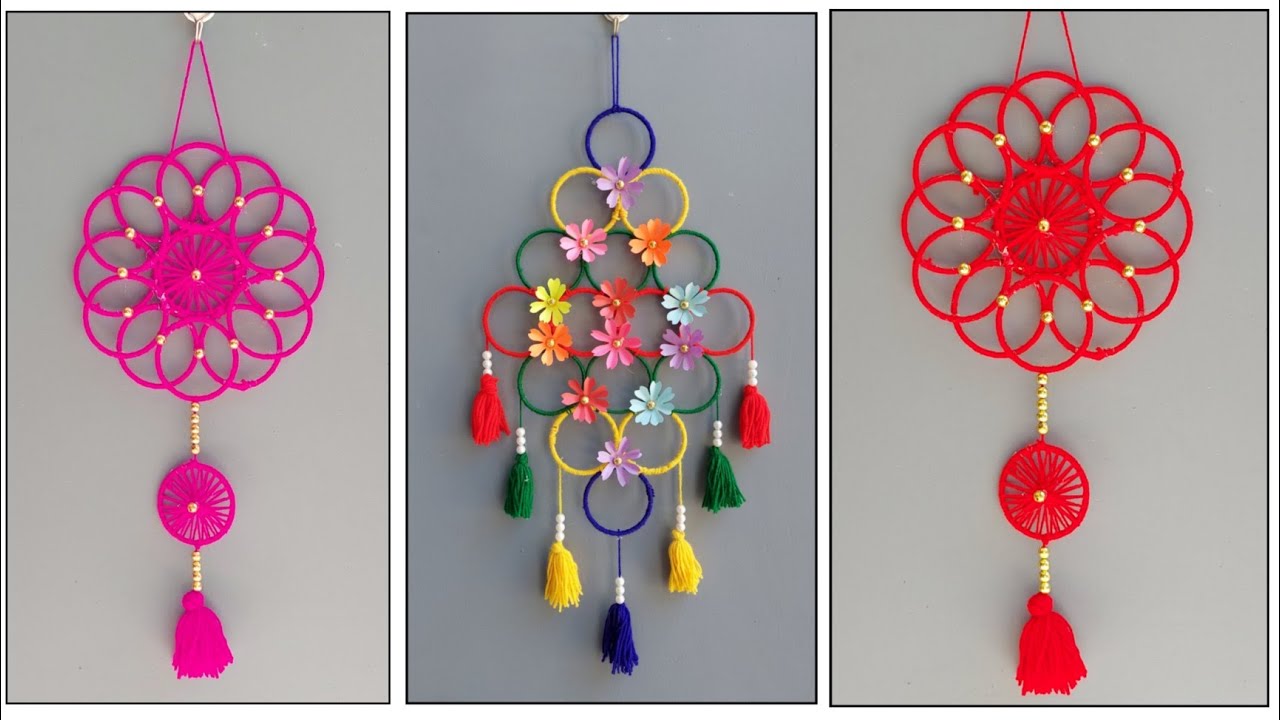The image showcases three intricately designed hanging art crafts, each suspended from strings against a light gray background. 

On the left side, a pink string supports a honeycomb-like flower-shaped structure composed of circular rings. Below this, a sequence of alternating white beads and pink circular objects leads to a bell-shaped puff at the end.

In the middle section, colorful interconnected rings are arranged in a pattern starting with a blue ring, followed by two yellow rings, three green rings, and four red rings. Below this arrangement, three green rings, two yellow rings, and one blue ring are accompanied by red, green, yellow, and blue puffs.

The right side features a red version of the floral honeycomb structure found on the left. This red object mirrors the pink one in shape and design, from the rings at the top to the patterned beads and the concluding bell-shaped puff.